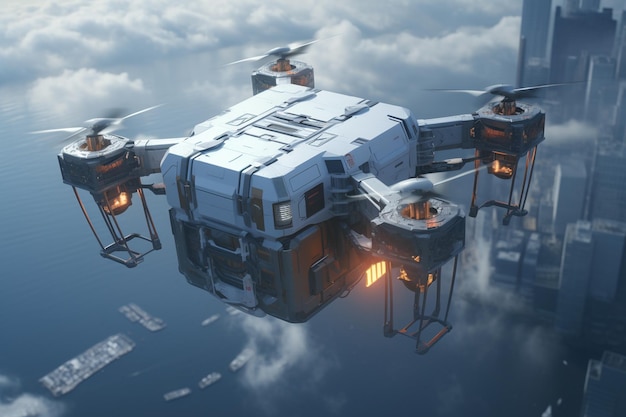The image depicts a digitally rendered, futuristic flying machine resembling a massive drone or a hybrid helicopter, with a prominent focus on its cargo-transporting capabilities. The central contraption has a cuboid shape characterized by a white top section and a metal and wooden lower half, suggesting a payload area designed to carry significant cargo or potentially passengers. It is supported by four large propellers attached to the corners, each mounted on dark gray square housings with cylindrical structures emitting an orange glow from the bottom, highlighting a high-tech, possibly AI-generated, design.

The scene is set high above a sprawling city, evident from the backdrop of towering skyscrapers made predominantly of glass, with notable tall buildings on the right-hand side. Below, a vast expanse of smooth, dark blue water is visible, dotted with what appear to be large ships or boats, lending an industrial and maritime ambiance to the setting. The sky around the vehicle features white clouds accentuated by dark blue hues, giving the entire composition a grayish-blue tone. The overall impression is that of an advanced, futuristic aerial vehicle navigating above a modern cityscape adjacent to a large body of water.